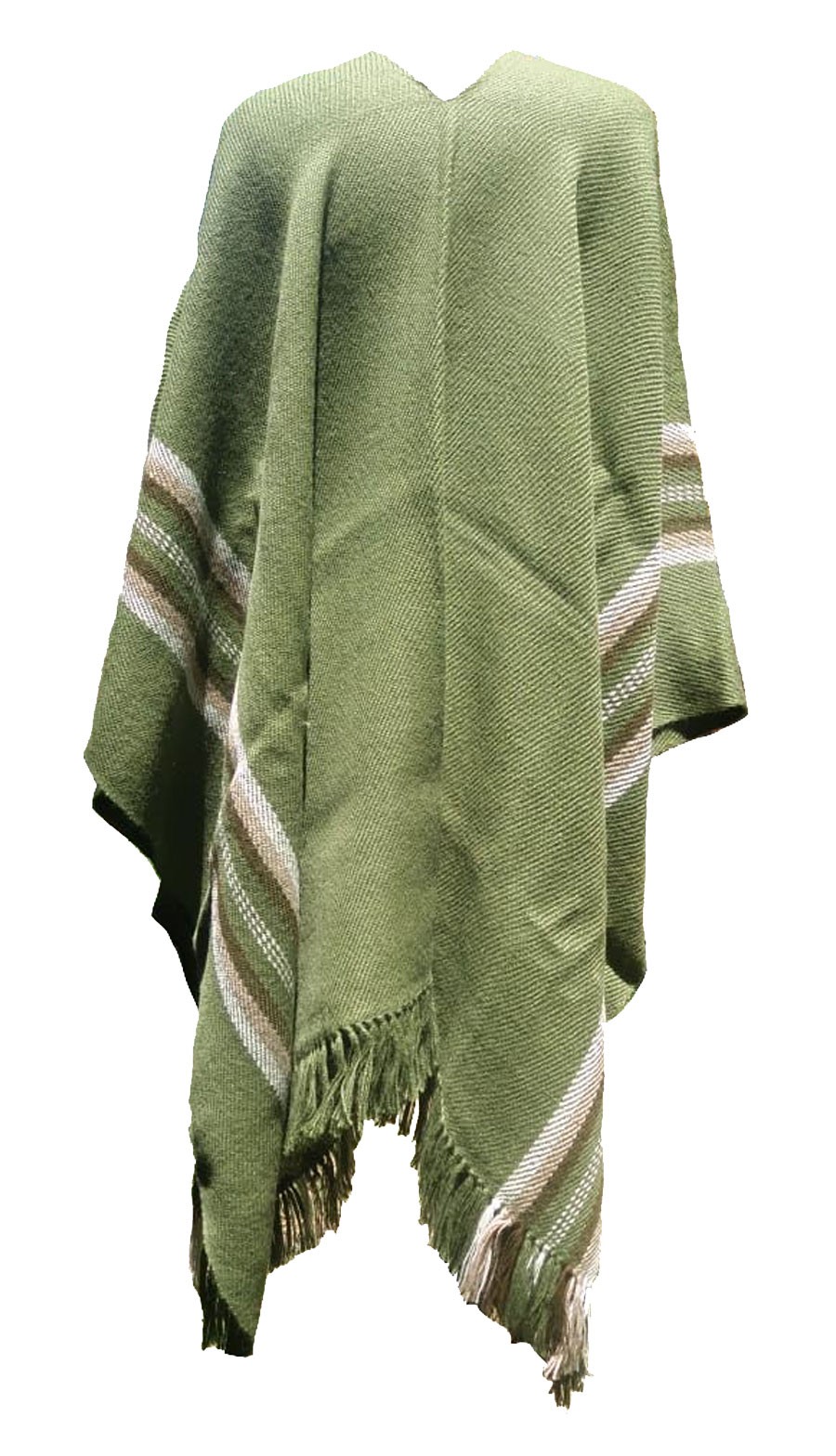This image features a sage, dusted olive green poncho, displayed against a white backdrop, appearing to float in the air. The poncho is made of a thick, textured, woven cloth and is draped over a form that hints at shoulder shapes. It has a v-neck cut for the head and unfolds into a large, flowing garment with a hem resembling a handkerchief. The poncho is accented with horizontal stripes towards the bottom, featuring a sequence of colors: white, tan, brown, variations of green, and a dashed white line. These stripes run from the front to back edges, which are free of fringe. The front and back, however, are adorned with long fringe matching the garment’s overall color scheme. The fringe and stripes lend detailed embellishment, complementing the predominantly mossy green hue of the poncho.